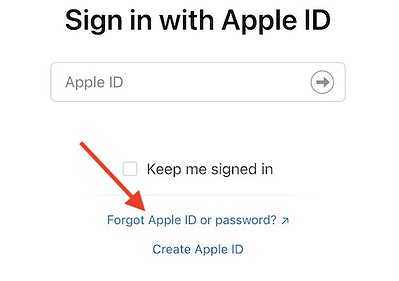The image is a screenshot from an application or web page designed for user authentication. The entire layout is set against a clean white background. At the top in bold black text, the title reads "Sign in with Apple ID." Below this, there is a gray-outlined box with the placeholder text "Apple ID" inside it, accompanied by a right-pointing gray arrow. Underneath the Apple ID input box, there is a checkbox next to the black text "Keep me signed in," which is currently unchecked. A faint gray line separates this section from the next.

Further down, a blue line of text reads "Forgot Apple ID or password" with a blue arrow pointing towards the top right corner, indicating it as a clickable link for users who need to recover their credentials. Just below this, in a slightly bolder blue text, the option "Create Apple ID" is available.

Additionally, a prominent red arrow is superimposed on the screenshot, directing attention specifically to the "Forgot Apple ID or password" link. Most of the primary text is in black, ensuring clarity, while placeholder text and certain secondary elements are in gray, maintaining a minimalist design.